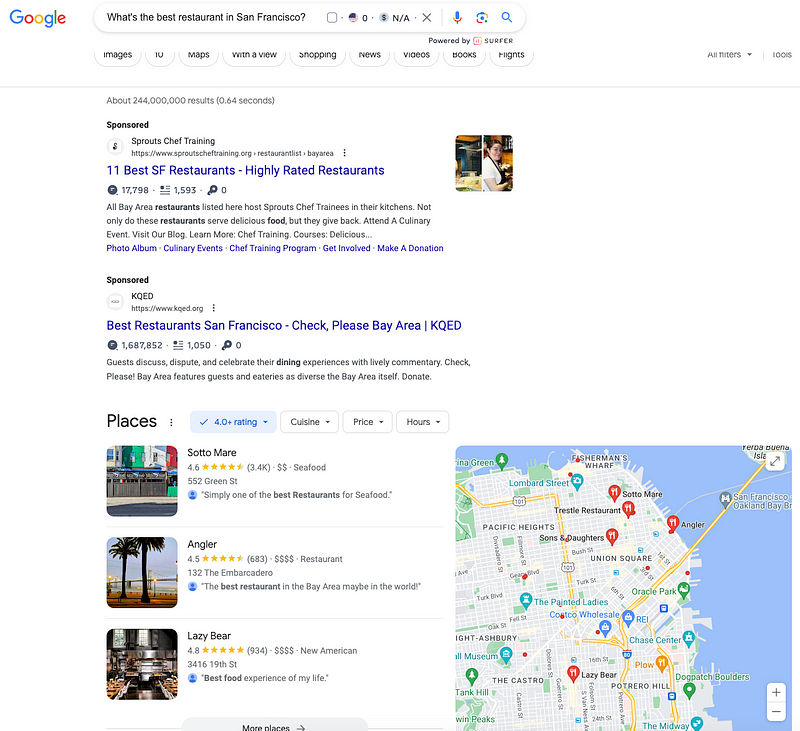The image is a screenshot of a Google search query for "best restaurant in San Francisco." The search results are organized in a visually informative manner. At the top, there are sponsored listings, the first of which suggests "11 Best San Francisco Restaurants, Highly Rated," followed by another sponsored link titled "Best Restaurants in San Francisco: Check, Please! Bay Area."

Beneath these, there are three notable restaurants prominently listed under the "Places" section: Sotto Mare, Angler, and Lazy Bear. On the right side of the screen, a detailed Google Map highlights the locations of these restaurants. The map extends to show a segment of the San Francisco Bay Area, encompassing neighborhoods such as Fisherman’s Wharf, the Castro, Haight-Ashbury, and Potrero Hill. Each of the listed restaurants is pinpointed, providing a clear visual reference for their locations.

Additionally, at the bottom of the "Places" listing, there is an option labeled "More places," indicating that further restaurant options can be viewed. Below the primary search result, there's a featured snippet for "Sprouts Chef Training," accompanied by an image of a young woman in a white shirt and apron, seemingly engaged in a culinary activity within a kitchen setting. The combination of search results and map provides a comprehensive guide for anyone seeking highly recommended dining options in San Francisco.